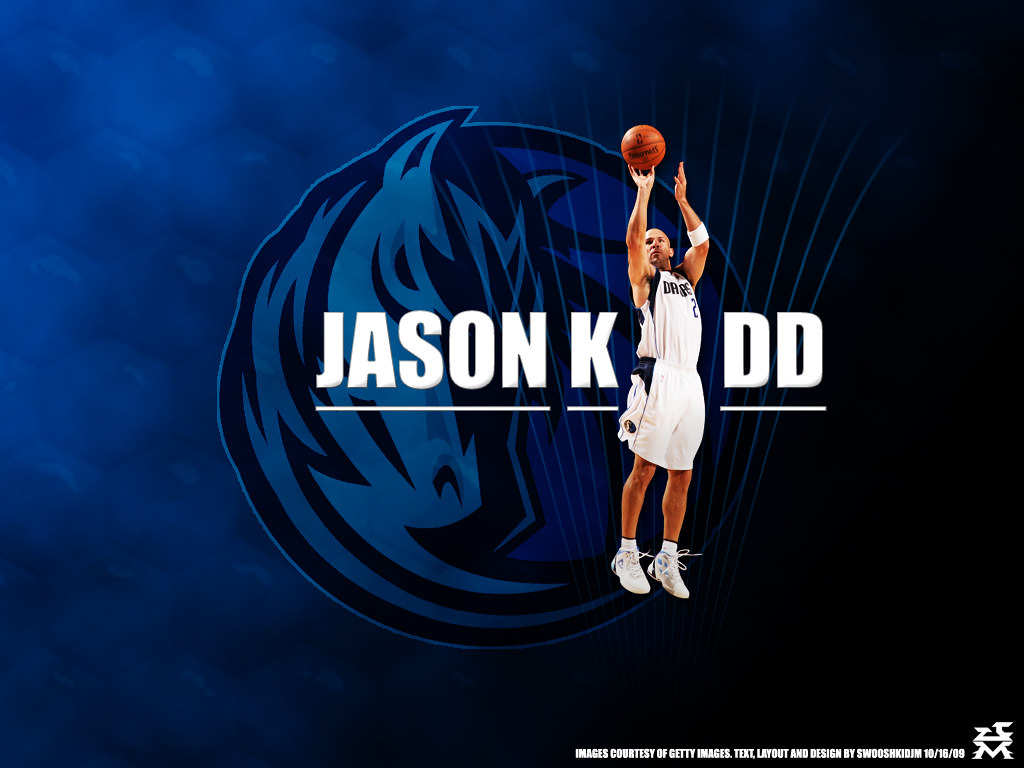The background of this image transitions seamlessly from black at the top to dark blue in the middle, fading into light blue at the bottom. Positioned centrally on the image is a translucent white logo of a horse, encased within a blue circle. Over this, bold, all-caps text in blocky letters reads "JASON KDD," meticulously underlined by a thin white line. Cleverly replacing the letter "I," which would normally appear between the first "K" and "D," is the figure of a basketball player in mid-action. This player, donning a white jersey and an armband, seems to be shooting a basketball. The text and design elements employ a palette of dark blue and black, harmonizing with the background. At the bottom of the image, a caption in smaller text reads "Images courtesy of Getty Images, text layout and design by SwooshKidJM101609."